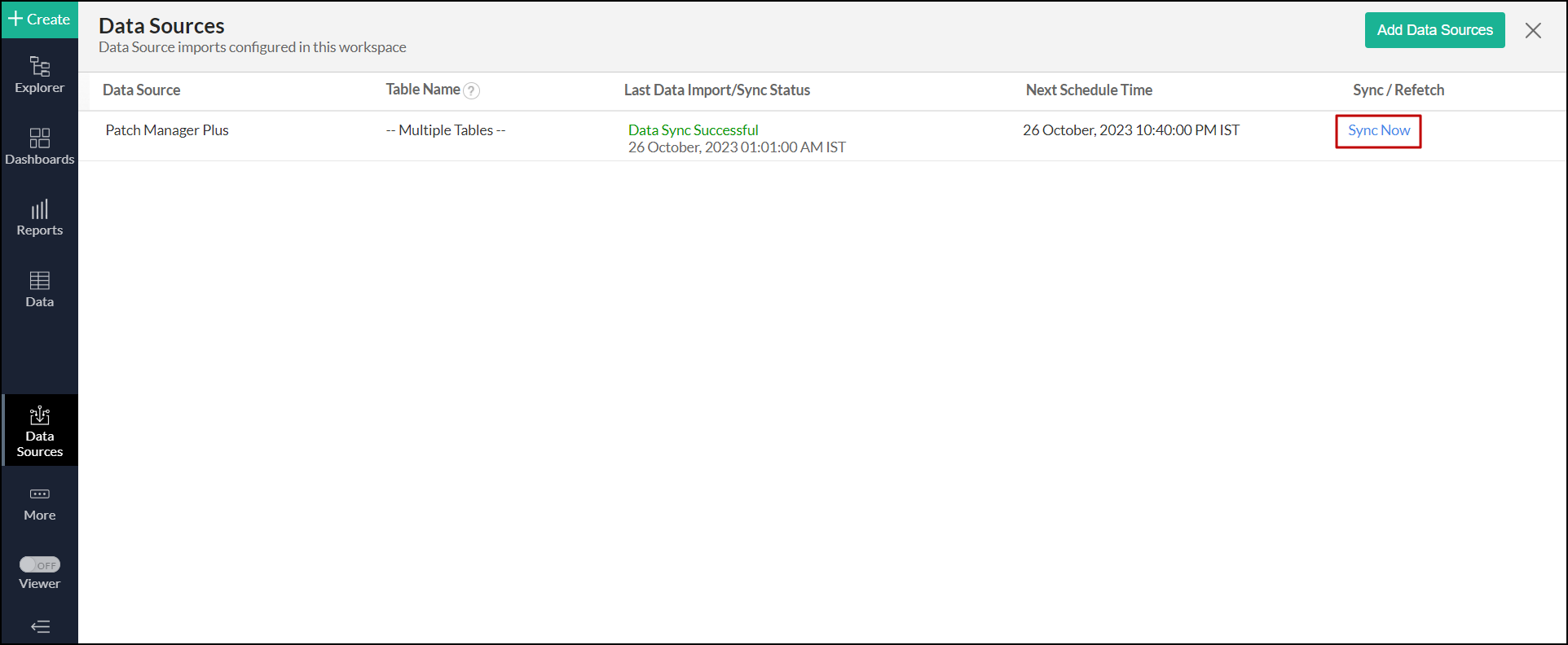The image presents an interface for managing data sources in a workspace. 

At the top, a bold black heading reads "Data Sources," followed by a subheading in smaller text stating "Data Source Imports Configured in this Workspace." On the top-right corner, there is a prominent green button with white text labeled "Add Data Sources," accompanied by an 'X' icon for closing the interface.

On the left side, a dark-colored navigation tab is visible. It features a green button labeled "Create" at the top, beneath which several options are listed in white text: "Explore," "Dashboards," "Reports," and "Data." The "Data Sources" option is highlighted in a darker color, indicating the current selection. Below these options, there is a "More" button followed by a toggle switch with the label "Viewer," set to "Off." Underneath this, a few lines with an arrow pointing to the left are displayed. Each option in the list is accompanied by a white icon.

The main section on the right displays a chart with a header that includes column titles: "Data Source," "Table Name," "Last Data Import/Sync Status," "Next Scheduled Time," and "Sync/Refetch." The first entry in the chart shows "Patch Manager Plus" under the "Data Source" column, "Multiple Tables" under "Table Name," "Data Sync Successful" along with a timestamp under "Last Data Import," another timestamp under "Next Scheduled Time," and a "Sync Now" button with a red outlined box under "Sync/Refetch."

The layout and structure of the interface are designed to facilitate easy navigation and management of data sources within the workspace.